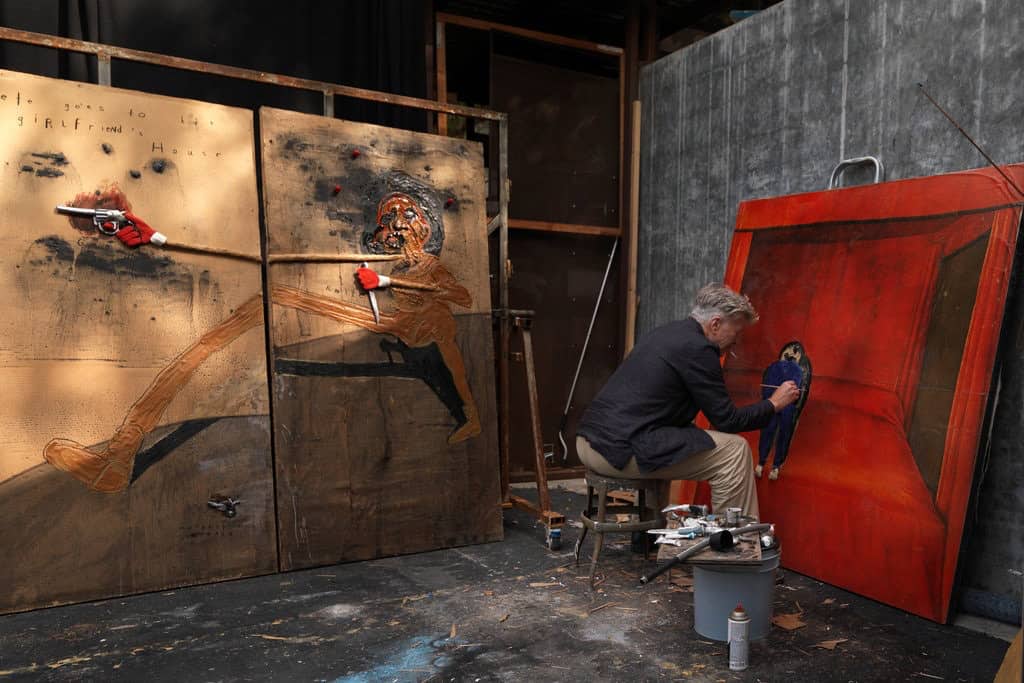In this image, a man is seated on a stool on the right side, engrossed in painting. He wears a dark-colored suit jacket paired with brown khaki trousers. With a paintbrush in his hand and another held in his mouth, he works diligently on a red canvas attached to a board. The red platform he paints on seems almost 3D, depicting what appears to be a humanoid structure or character on the canvas. To his side, various tools are scattered, including a smaller wooden board perched atop a gray bucket and spray paint cans with red tips. Behind him, the wall displays additional artworks, including a caricature of a person with exaggeratedly stretched limbs and a gun. The environment exudes the organized chaos of an artist's studio. The man might also be smoking a cigarette, which hangs loosely from his mouth as he paints.